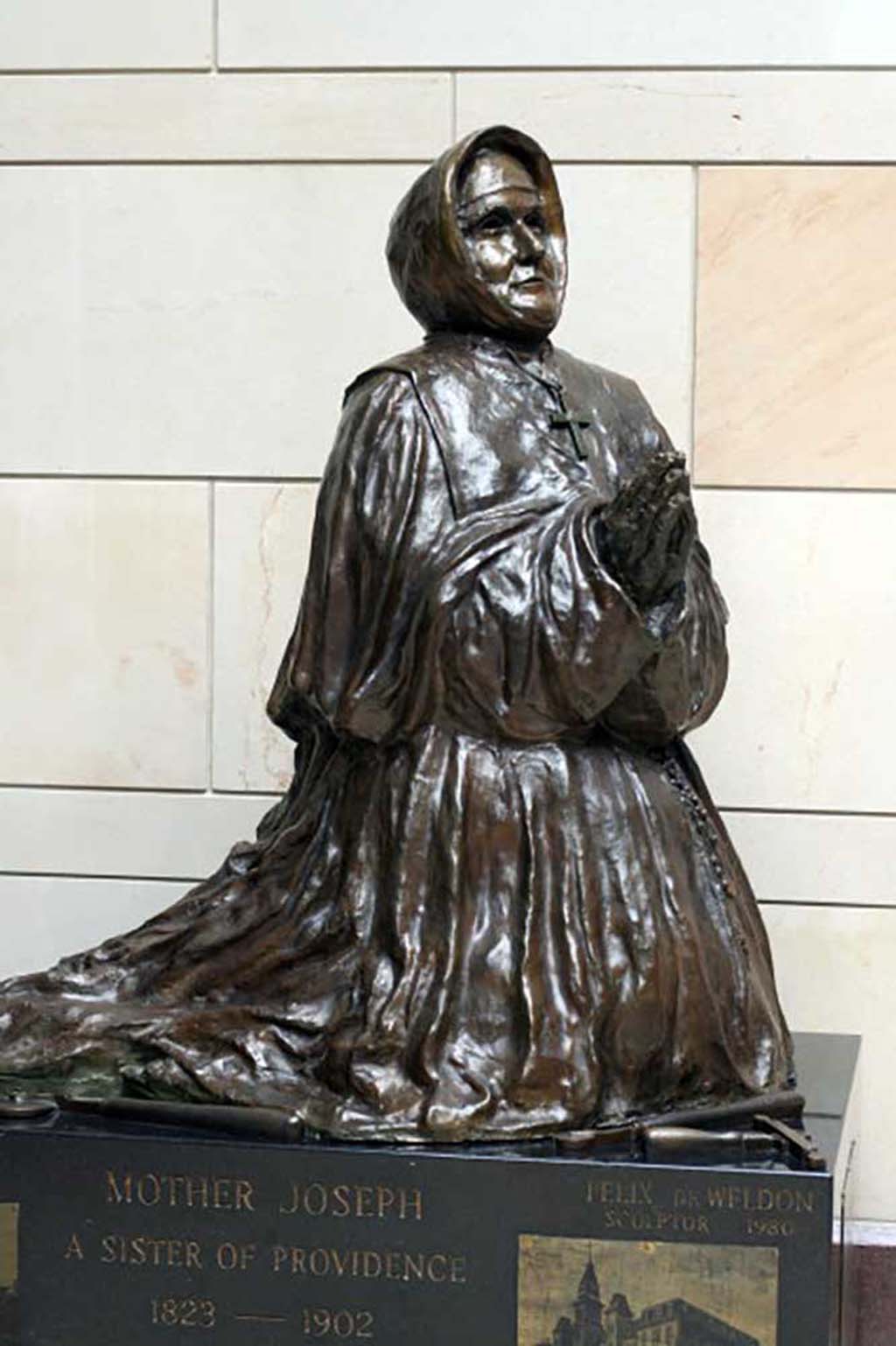In this striking image, a bronze statue of Mother Joseph, a revered Sister of Providence, stands prominently against a large block wall. Cast in dark, richly patinated bronze, Mother Joseph is depicted in a posture of deep prayer, kneeling with her hands clasped earnestly. Her nun's habit, meticulously detailed, drapes gracefully around her, with the fabric of her skirt noticeably gathered where it meets the ground. A large cross hangs around her neck, embodying her devout faith. At the base of the statue, an inscribed plaque provides context, featuring a depiction of a church and affirming her identity and significance. Beside the statue, a contrasting red block adds a vibrant touch to the scene, emphasizing the reverent atmosphere surrounding this homage to Mother Joseph's legacy.